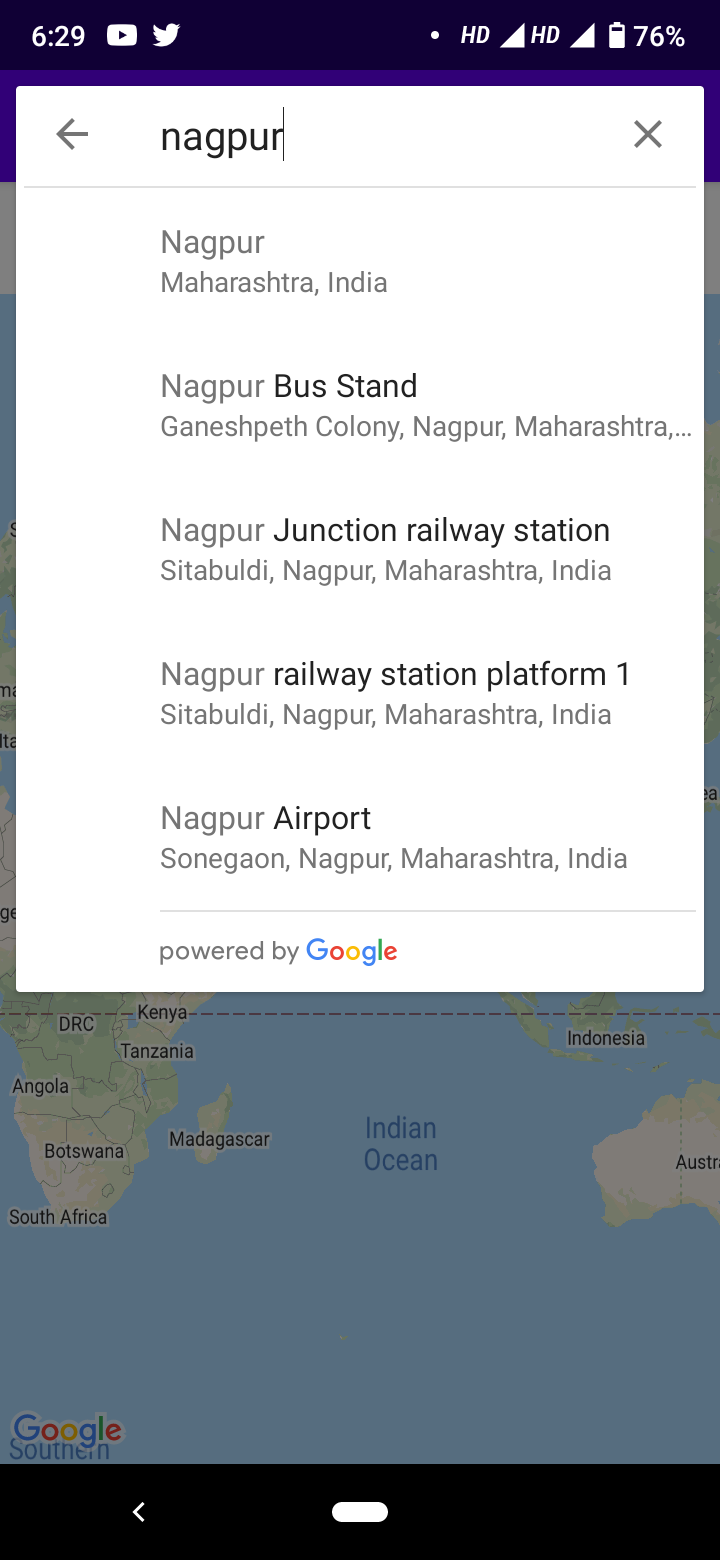Screenshot of a mobile phone displaying a map of India. A pop-up menu overlays the map, featuring an input text box with "N-A-G-P-U-R" entered. Beneath the input box, the search results list:

1. Nagpur in Maharashtra, India
2. Nagpur Bus Stand in Ganeshpur Geth Colony
3. Nagpur Junction Railway Station
4. Nagpur Railway Station Platform 1
5. Nagpur Airport

The time displayed on the phone screen is 6:29.